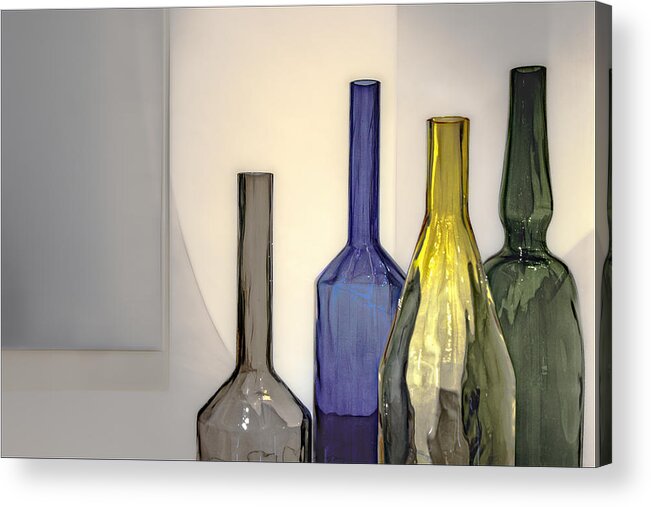The painting depicts four glass bottles arranged against a predominantly white background, imbued with subtle shades of light gray and a hint of blue. From left to right, the bottles are a clear grayish one, a blue one, a yellow one, and a grayish-green one. The grayish-green bottle, the tallest among them, is the widest as well, though the yellow bottle, standing in front of it, partially obscures its view. The blue bottle, slightly taller than the yellow one but shorter than the greenish one, features a long neck and stands subtly behind the yellow bottle. The yellow bottle, characterized by its shorter stem, does not rival the height of the others but stands prominent due to its vivid color. The clear gray bottle on the far left is the shortest, with a long stem and a shiny finish, giving it an almost black appearance. None of the bottles share the same height, creating an asymmetrical yet harmonious arrangement that casts dynamic shadows on the background. The composition primarily directs focus towards the bottles placed more towards the right side of the canvas, accentuating their unique features and colors amidst the pale backdrop.